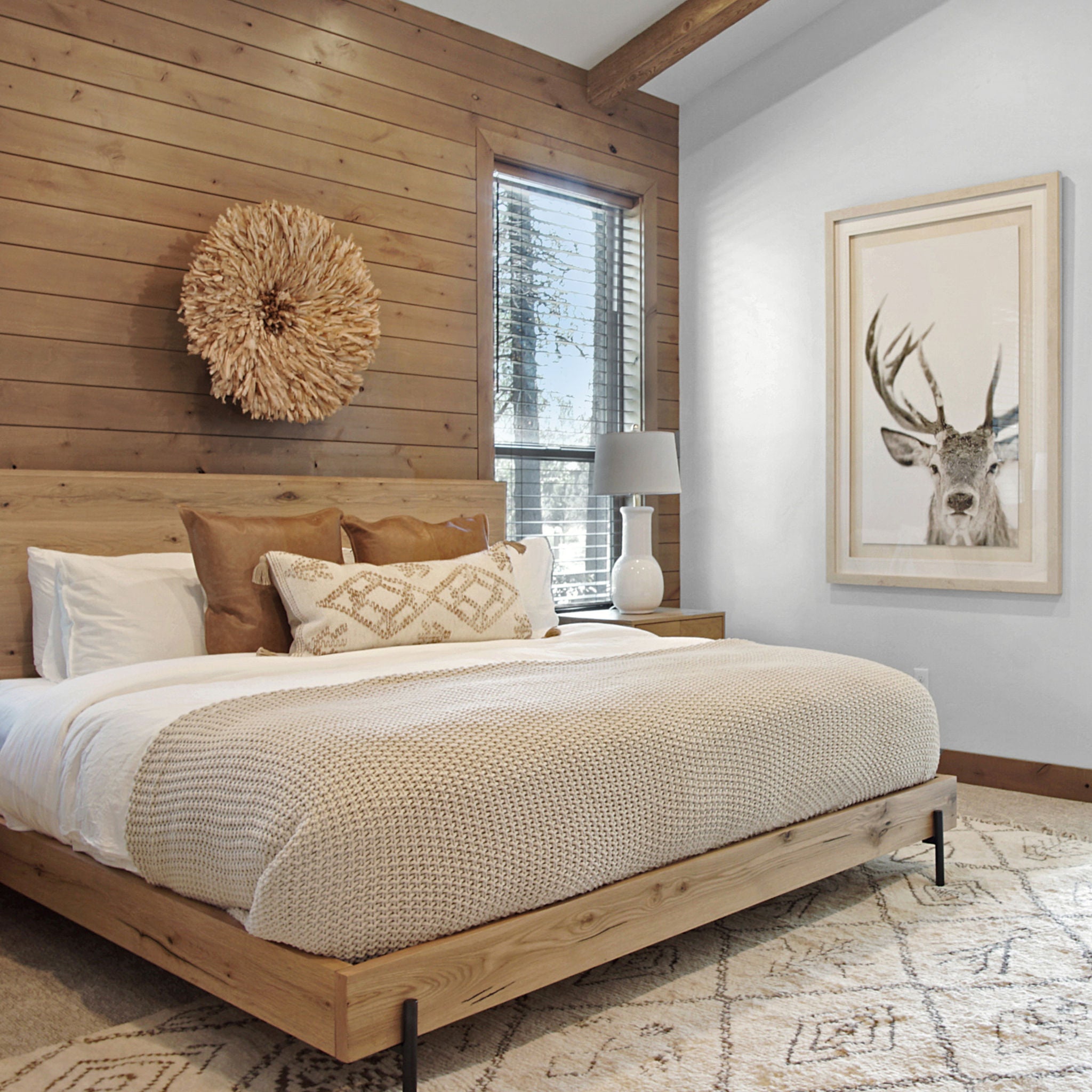The photograph showcases a cozy bedroom adorned with earth tones and a rustic aesthetic. The focal point of the room is the wooden bed frame with black metal legs, featuring a wooden headboard. The bed is dressed in light beige sheets, a matching comforter, and layered with various pillows, including two white pillows, two brown cushions, and a distinctive long pillow with tassels and a diamond-patterned pillowcase. The wooden paneled wall behind the bed is decorated with a large flower sculpture, adding a touch of artistry to the space.

On the floor, there is a light brown carpet partially overlaid with a patterned rug featuring diamond shapes and symbols, adding texture and interest to the flooring. A brown bedside table sits next to the bed, holding a white lamp that softly illuminates the area. An open window, adorned with blinds, allows natural light to stream in and provides a view of the surrounding trees.

Additionally, the room features white walls and ceiling with wooden molding at the bottom, complementing the rustic theme. Opposite the bed, a large framed painting of a buck or deer in brown and tan tones further enhances the earthy color palette and the natural, serene ambiance of the bedroom.